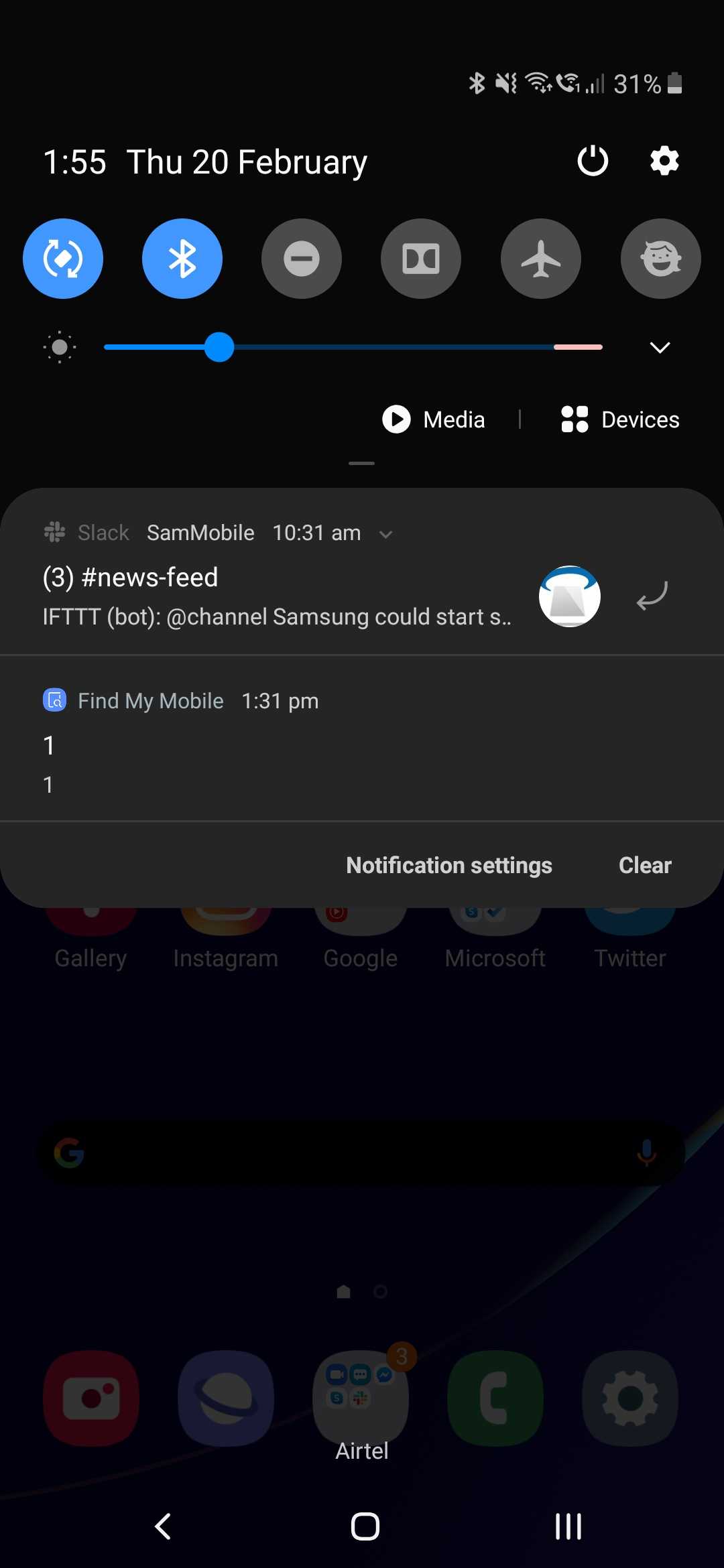Screenshot of a phone display showcasing the status and notification bar at the top, where we can clearly see multiple icons: Bluetooth, sound set to vibrate, Wi-Fi, phone call, and signal strength at two bars. The battery level is at 31%. The date and time are displayed below these icons, indicating it is Thursday, February 20th, at 1:55 PM.

Further down, two phone icons, highlighted in blue, show the selected options for screen toggling and Bluetooth connectivity. The brightness bar is just below these, set at a little less than half brightness. Below this, there is a section for 'Media and Devices,' followed by notification boxes for Slack and SamMobile. The Slack notification indicates there are three messages in the #newsfeed channel, sent at 10:31 AM.